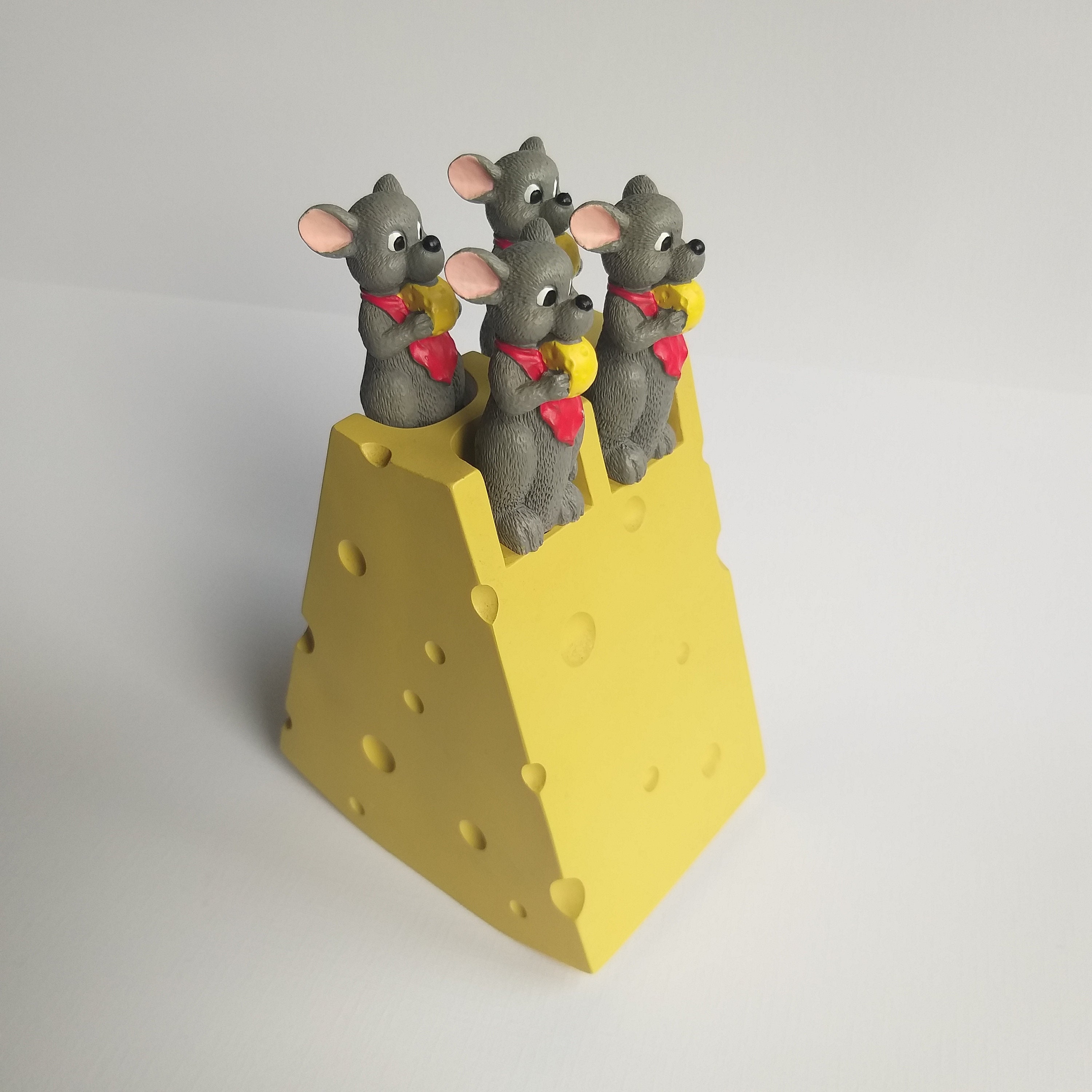This photograph features a whimsical child's toy positioned against a clean, white background with subtle shadows. At the center of this square image sits a large, wedge-shaped block of yellow plastic cheese, resembling a classic piece of Swiss cheese with holes. The wider base of the cheese wedge is placed at the bottom, tapering up to the pointed tip. Atop this simulated cheese are four endearing gray mice figurines, each nestled into recesses on the cheese's surface, as if they have nibbled their way into it.

Each mouse is identical in design: they have round, gray bodies with prominent, pink inner ears, expressive black and white eyes, and tiny black noses. All four mice are equipped with vibrant red bibs that cascade down to their bellies, giving them an appearance of tidiness as they feast. These delightful characters, two positioned at the front and two at the back, are all grasping a piece of cheese with their little arms and appear to be in the middle of a shared meal, adding a narrative charm to the scene.

The overall set-up of the image, with its pristine, undistracted backdrop, suggests an intentional display, akin to a product photograph designed for online marketplaces like eBay. The attention to detail in both the toy and the image composition highlights the playful creativity and inviting simplicity of this charming children's toy.